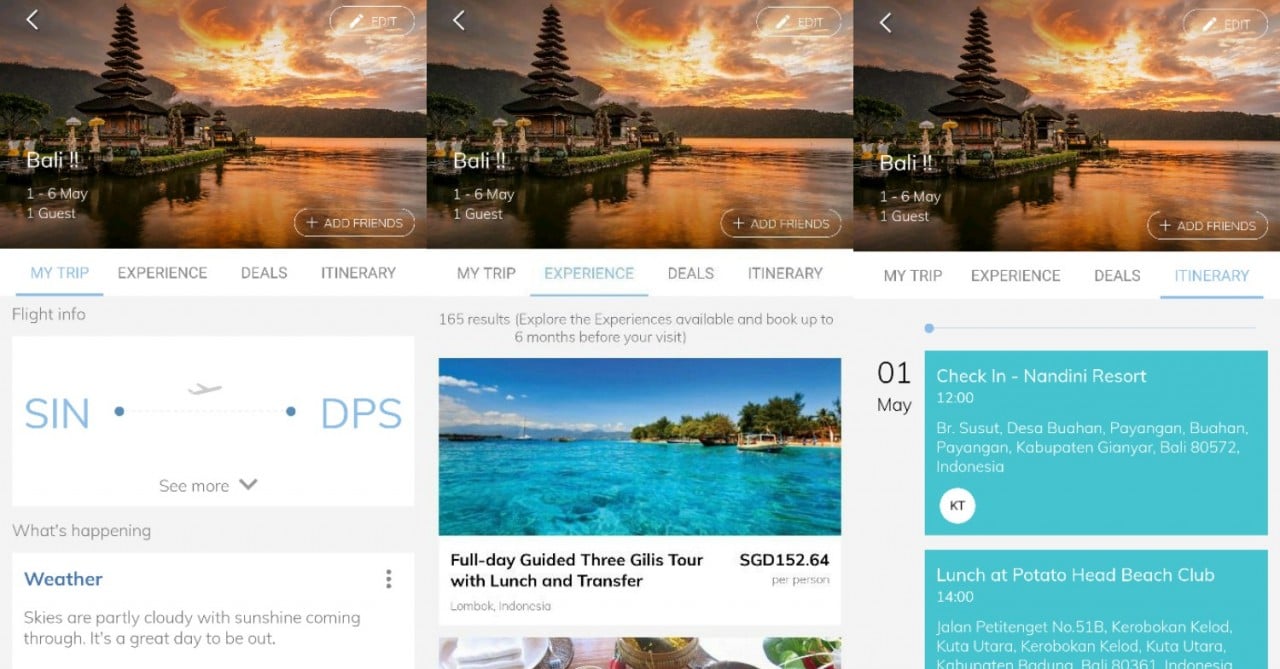The image depicts a three-section webpage interface related to travel booking, likely the itinerary page for a trip to Bali from May 1st to May 6th for one guest. The overall layout of the webpage extends to double its height, with each section equally sized.

At the top, occupying about 35% of the vertical space, is a stunning banner featuring a picturesque scene of either a sunrise or sunset. The sky is illuminated with vibrant hues of purples, oranges, and yellows, partially hiding behind clouds. In the distance, shaded mountains cast dark silhouettes, almost black, against the colorful sky. The sunlight reflects off a body of water in the foreground, adding to the tranquil atmosphere. On the left side of the water, a dock is visible, enhancing the scenic beauty.

The header text on the left side of the banner reads: "Bali, 1-6 May, 1 Guest," indicative of the trip details being viewed or booked.

Below the banner, the three navigation menus are displayed horizontally. The first menu labeled “My Trip” on the left is highlighted in blue, indicating it is the current section viewed. The second menu item, “Experience,” is also highlighted in blue. The third menu item, "Deals," remains unhighlighted. The final menu item, “Itinerary,” on the far right, is also highlighted in blue, suggesting active engagement with these sections.

Within the content areas of each section:
- The left section titled “My Trip” displays various destinations.
- The center section, labeled “Experience,” shows beautiful images likely intended to entice the traveler.
- The right section under “Itinerary” provides a detailed schedule, outlining the plans and activities for the trip.

Overall, the webpage excels in balancing aesthetic appeal and functional design, aiming to provide a seamless booking experience for the traveler.